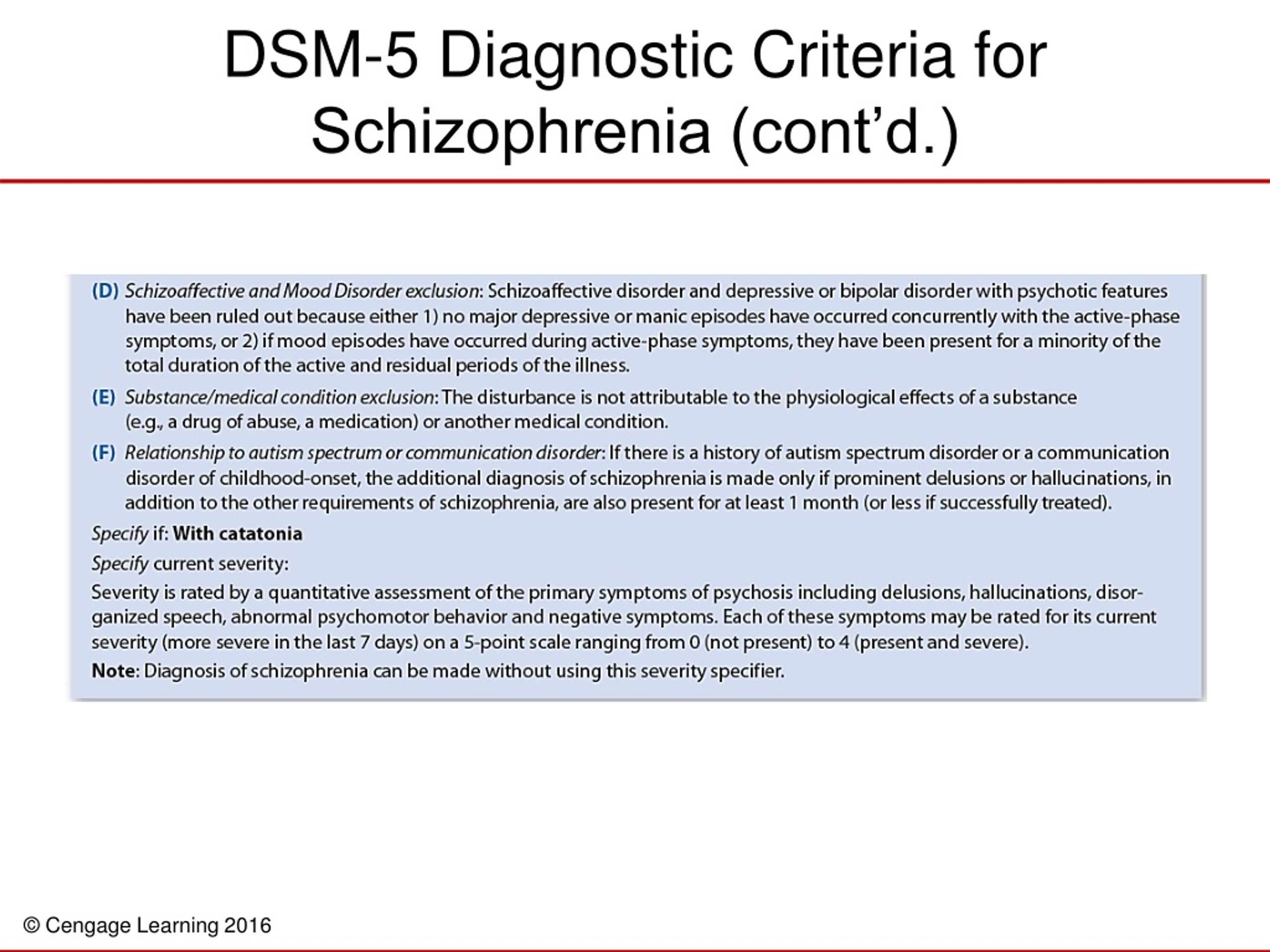The image depicts a webpage featuring diagnostic criteria from the DSM-5 for Schizophrenia. The webpage has a predominantly white background with black, red, and blue text. At the top of the page, in large font, it reads "DSM-5: Diagnostic Criteria for Schizophrenia" with a note indicating continuation in brackets. A red line separates the header from the main content of the article below. 

The main content includes a blue rectangular box with black text, categorized by letters D, E, and F, each in blue font. Section D, titled "Schizoaffective and Mood Disorder Exclusion," details the criteria for ruling out schizoaffective disorder and depressive or bipolar disorder with psychotic features. The text explains that these mood disorders are excluded either if no major depressive or manic episodes occur simultaneously with the active phase symptoms, or if such mood episodes are present, they occur for a minority of the total duration of the active and residual illness periods.

Section E addresses "Substance/Medical Condition Exclusions," though the specific content for this part is not fully visible in the image.